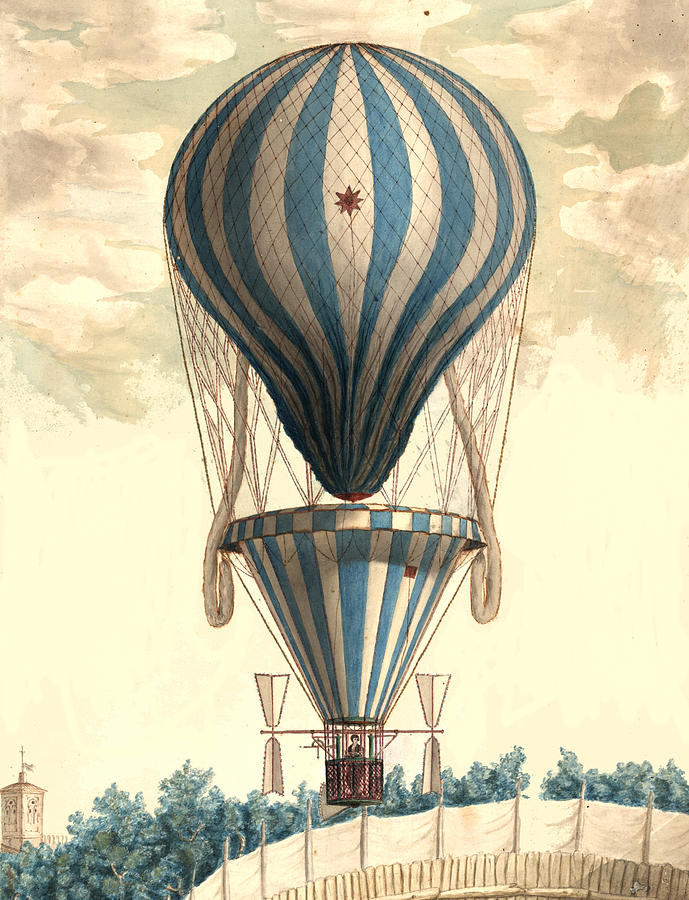The image is a detailed cartoon graphic created by an artist, depicting an old-fashioned hot air balloon soaring above a park-like area. The balloon itself is central in the composition and is large, with distinct blue and white stripes. A red star is noticeable in the middle of the balloon. Below the balloon is a giant, cone-shaped structure tied to it, and underneath this cone hangs a small cylindrical basket holding a single person, presumed to be the conductor. The basket is surrounded by green and red netting with additional parts that stick out. The style of the artwork, possibly done in watercolors or colored pencils, gives it an old-timey feel, enhanced by cream-colored and greenish-gray clouds partially obscuring the sun at the top of the image. In the background, the scene is completed with depictions of trees and a hint of a building's top in the bottom left corner, indicating the balloon is aloft and not grounded.